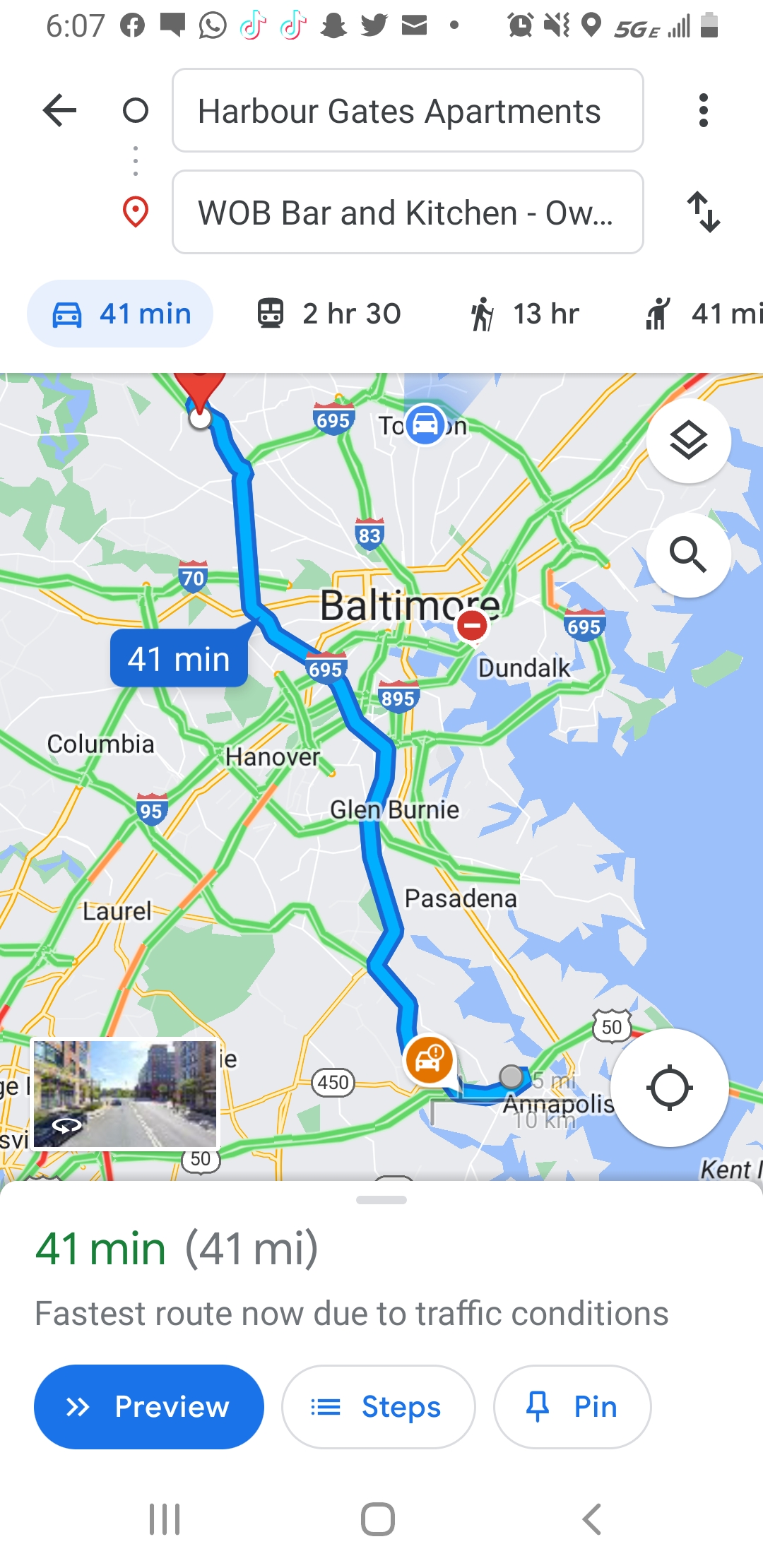This image is a detailed screenshot of a phone displaying a Google Maps navigation screen. At the top of the screen, you see standard phone icons: the time is 6:07, with app icons for Facebook, a speech bubble, a phone, TikTok, Snapchat, and Twitter to the left. There's also a 5G logo, a signal bar, and a battery life icon. The map itself shows a route between Harbor Gates Apartments and WOB Bar and Kitchen in Baltimore, Maryland. The route is highlighted in a thick blue line, predominantly running north to south, then slightly southeast to northwest. Secondary roads are displayed in white, with highways such as 695 in medium blue outlined in darker blue. Additionally, some roads are color-coded green, yellow, and orange, possibly indicating traffic conditions. At the bottom of the screen, there's a time estimate of 41 minutes and a distance of 41 miles for the route. The map also shows cities around Baltimore, including Columbia, Hanover, Dunlop, Renfrew, Pasadena, and Annapolis, with lesser highways in green and yellow. In the lower left of the map, there’s a small photo as well.